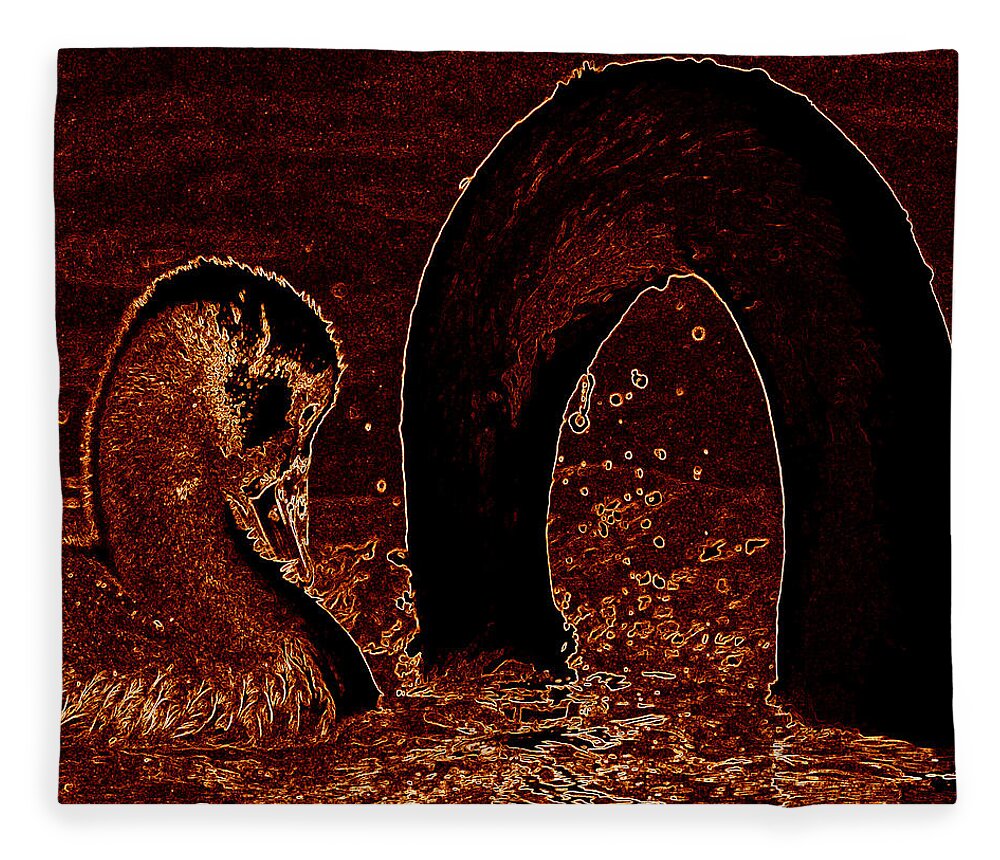The artwork is a dark, abstract piece dominated by shades of red, black, and rust with accents of white. The central figure appears to be a duck swimming through water, distinguished by its rust-colored body and black accents with its head tucked close to its bill. The water depicted is rough, textured with numerous small squares and white streaks giving a sense of fluid motion. The background is a deep red merging into black, reminiscent of a wood grain pattern. A prominent feature within this piece is a black archway, bordered by white lines, resembling a horseshoe shape that encapsulates the red and white elements of the scene. This art could be either an oil painting or a heavily manipulated photograph, adding to its enigmatic presence. The overall composition is set within a square frame emphasizing the dark, almost burgundy tones contrasted by hints of golden beige and white. The black archway gives an impression of a sea monster or eel-like form, contributing to the mystique and peculiar charm of the artwork.